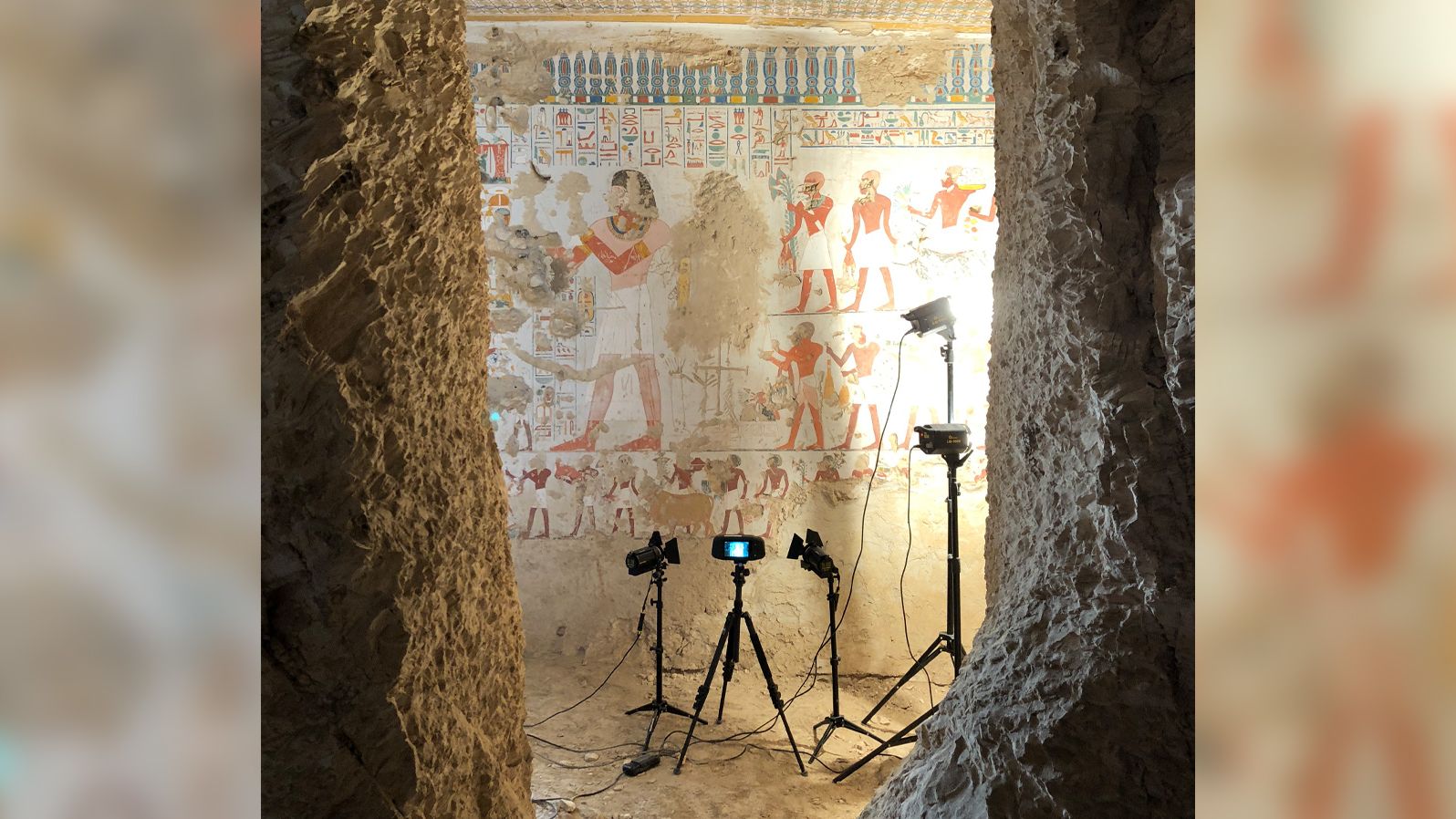The photograph captures the interior of an ancient Egyptian tomb or cave, its walls adorned with faded hieroglyphics and depictions of figures dressed in white kilts. The walls, primarily tan in color with touches of reddish-brown and blue, bear the marks of age. The scene is meticulously documented by five black cameras perched on tripods, surrounded by ancillary film and lighting equipment. The image, taken from an adjacent room through a hole in the wall, reveals a setup likely for archaeological documentation or perhaps a film production. Dirt and stone pillars or columns make up the foreground, emphasizing the historical and archaeological significance of the site.